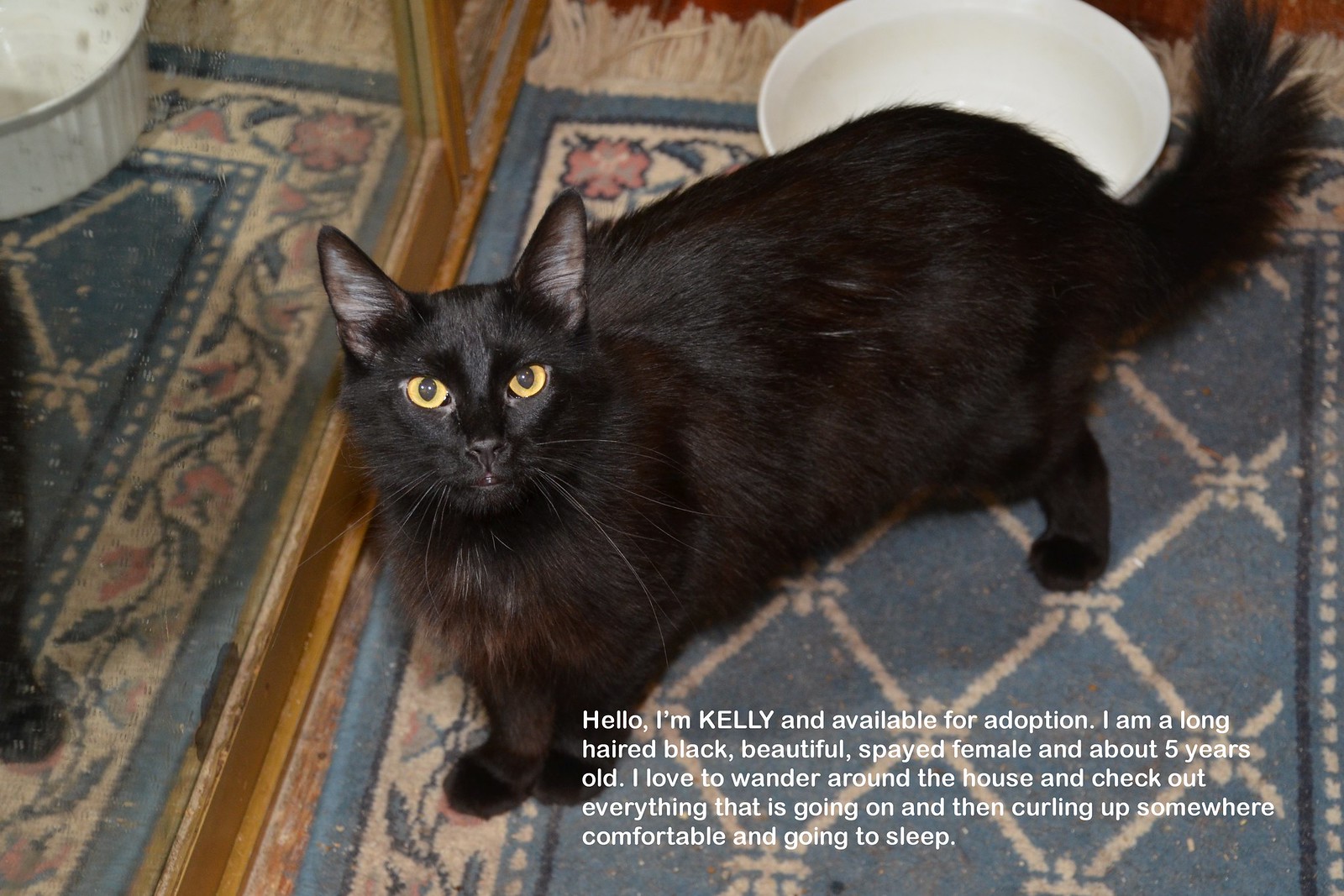The horizontally rectangular, full-color promotional photograph features a beautiful long-haired black cat with striking yellow eyes. The cat is positioned on a blue rug with white crisscross patterns, standing in front of a closet mirror that reflects its surroundings. While the cat's body faces left in a side profile, its head is turned to gaze directly into the camera. To the right of the cat is a white bowl that appears similar to a baking dish. At the bottom of the image is white text that reads, "Hello, I'm Kelly and available for adoption. I'm a long-haired, black, beautiful spayed female and about five years old. I love to wander around the house and check out everything that's going on and then curl up somewhere comfortable and go to sleep." The image serves as an advertisement for pet adoption, capturing Kelly's appealing features and inviting potential adopters to bring her home.